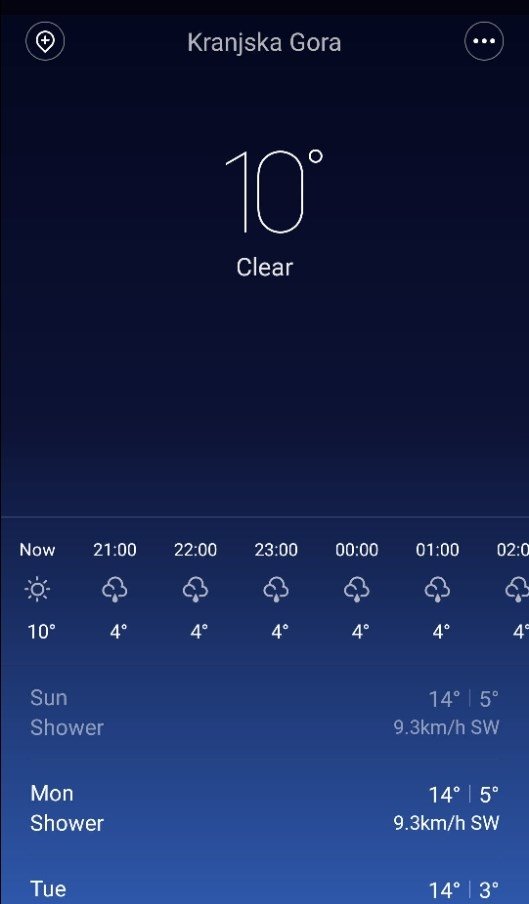Screenshot of a Weather App Interface in Portrait Mode

The screenshot appears to be taken from a weather application on a mobile device displayed in portrait mode. The background gradient transitions from almost black at the top to a deep blue towards the bottom. 

- **Top Section**: 
  - Upper left corner features an icon resembling a pointer with a plus symbol.
  - Centered at the top, the text "Kranjica Gora" is displayed, suggesting the name of the location, likely a town or city.
  - Upper right corner features a three-dot menu icon.

- **Middle Section**: 
  - Centrally placed, large white text reads "10°", with the word "Clear" directly under it in a slightly smaller font.

- **Hourly Forecast Section**: 
  - Occupying roughly the middle third of the screen, this section lists times running horizontally from "Now" through 21:00, 22:00, 23:00, 00:00, 01:00, and 02:00 hours.
  - Each time slot provides weather details: 
    - "Now" displays a sunny icon and "10°".
    - The subsequent time slots show a cloud with a single raindrop icon and a temperature drop to "4°".

- **Additional Weather Details Section**: 
  - Below the hourly forecast, there is a section providing more detailed weather conditions.
    - On the left, icons for "Sun" and "Shower" are present.
    - To the right of these icons, temperature readings are shown, along with wind speed in kilometers per hour and direction.

- **Daily Forecast Section**: 
  - Further down, this section features a stack of columns labeled "M O N" (presumably for Monday) and "Shower."
  - The right side continues with similar details: temperature, weather conditions, and wind information.
  - At the very bottom, the section begins with "TUE," indicating Tuesday, along with degree settings and rain forecasts extending to the far right.

The screenshot provides a comprehensive view of current weather conditions, an hourly forecast, and additional parameters such as wind speed and direction, tailored for the location "Kranjica Gora."